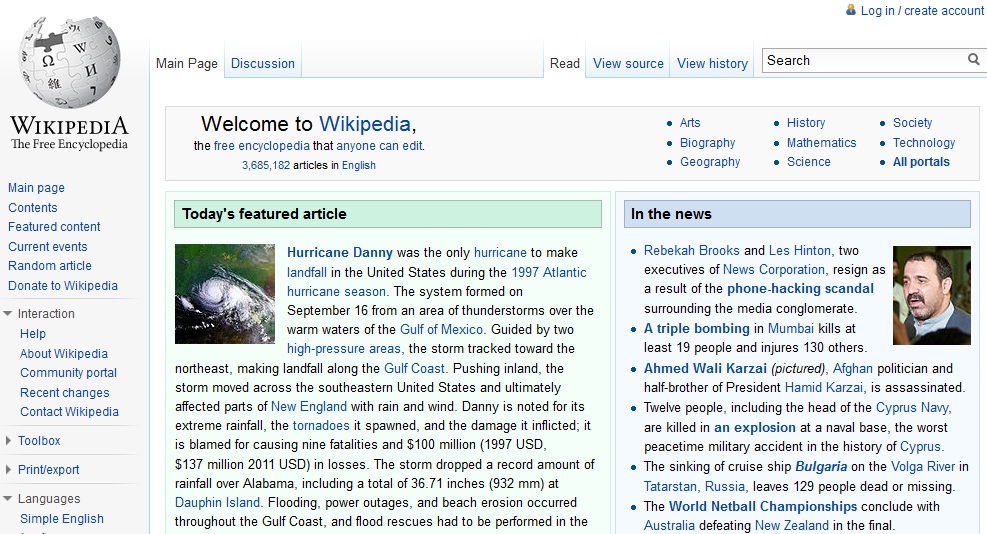This is a detailed screenshot of a Wikipedia page. On the left side is the iconic Wikipedia logo: a large, globe-like structure open at the top, composed of interlocking puzzle pieces adorned with various letters and symbols from different writing systems. Beneath this emblem, the text reads, "Wikipedia, the free encyclopedia."

Running down the left sidebar in blue lettering are navigation links, including: "Main Page," "Contents," "Featured Content," "Current Events," "Random Article," "Donate to Wikipedia," "Interaction," "Help," "About Wikipedia," "Community Portal," "Recent Changes," "Contact Wikipedia," "Toolbox," "Print/Export," and "Languages," with "Simple English" as one of the options.

At the top of the page, spanning horizontally, is a grey banner that announces, "Welcome to Wikipedia, the free encyclopedia that anyone can edit," highlighting the platform's inclusivity. The banner also notes, "3,685,182 articles in English."

On the right-hand side, there are bulleted lists organizing the content into categories: "Arts," "Biography," "Geography," "History," "Mathematics," "Science," "Society," "Technology," and "All Portals."

Further down on the left, a green banner marks the section titled "Today's Featured Article." On the right, a blue banner designates the "In the News" section. Both banners highlight current and significant content, keeping readers informed and engaged.